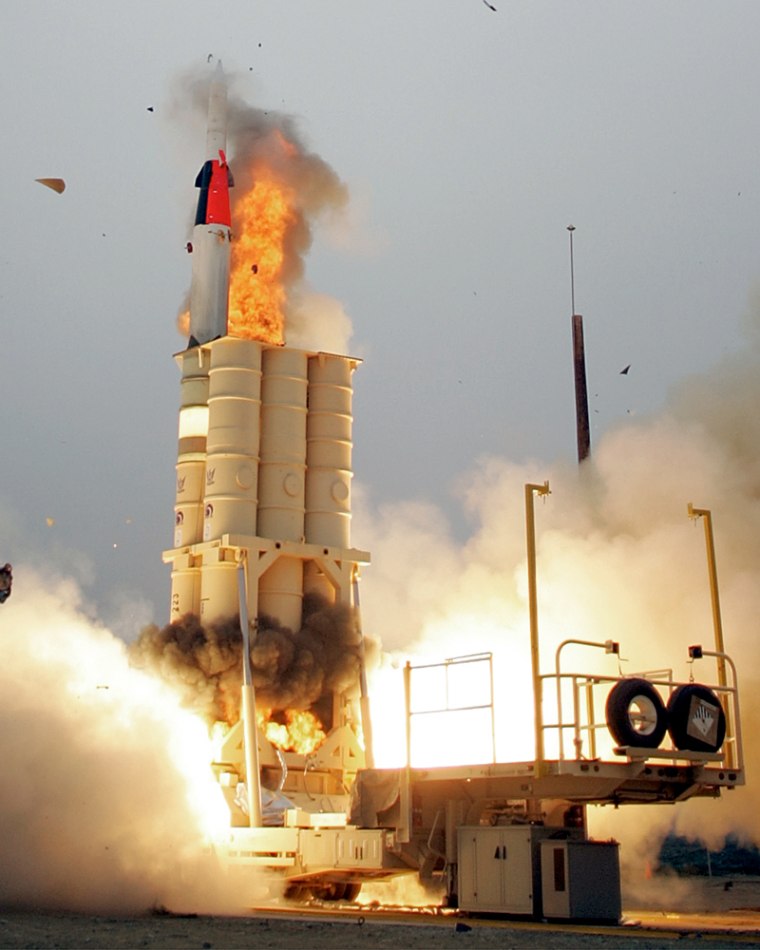In this photograph, we observe what appears to be a NASA-related scene, featuring a launch platform potentially used for rockets or spaceships. Central to the image is a small rocket component adorned in red and black, positioned amidst significant mechanical infrastructure. The rocket or missile is flanked by six cylindrical pipes, from which flames and thick, gray smoke are emanating. Below these pipes, more flames and unburned fuel or soot are visibly rising. 

Foreground details include two black tires mounted on a platform, with arching structures extending upwards. The environment is veiled in dense smoke, contributing to a hazy, gray sky backdrop. This expansive area, brightly lit but shrouded in smoke, suggests ongoing combustion and possibly a launch sequence. The overall scene is indicative of intense mechanical activity, likely tied to rocket or space shuttle operations, creating a vivid and dramatic depiction of aerospace engineering in action.